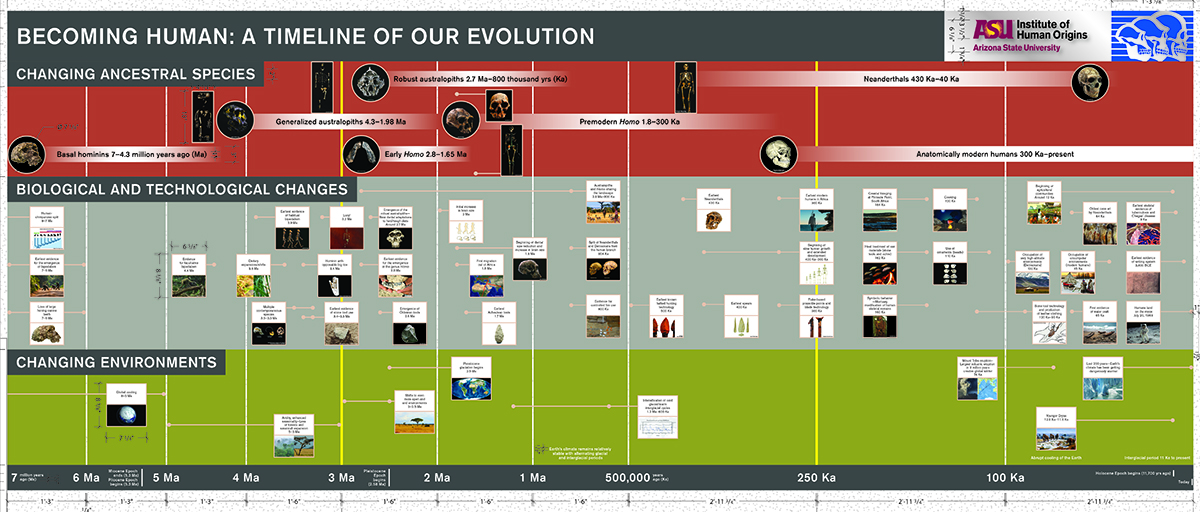The image is a detailed timeline titled "Becoming Human: A Timeline of Our Evolution," presented by the Institute of Human Origins at Arizona State University. It is divided into three horizontal sections, each marked by distinct colors: red, gray, and olive green.

The top section, with a red background, is labeled "Changing Ancestral Species." This segment provides a chronological account of the evolution of various ancestral species, starting from approximately 7 to 6.3 million years ago. Although the specific details are hard to discern, this section likely traces early hominids, including mentions of Australopithecus and other significant early ancestors.

Beneath this, the middle section features a light gray background. It highlights "Biological and Technological Changes" and maps out key developments over time. This part of the timeline illustrates how biological and technological advancements influenced human evolution, represented by various icons and images.

The bottom section, with an olive green background, details "Changing Environments." It includes text and images that explain how environmental shifts have played crucial roles in the evolutionary process.

The timeline is meticulously segmented into various time frames, with labels indicating periods such as 7 million years ago, 6 million, 5 million, and so on, down to recent history. As the timeline approaches the present day, the intervals become smaller, initially decreasing by millions of years, then by 500,000 years, 250,000 years, and finally by 100,000 years, reflecting more detailed evolutionary changes in more recent periods.